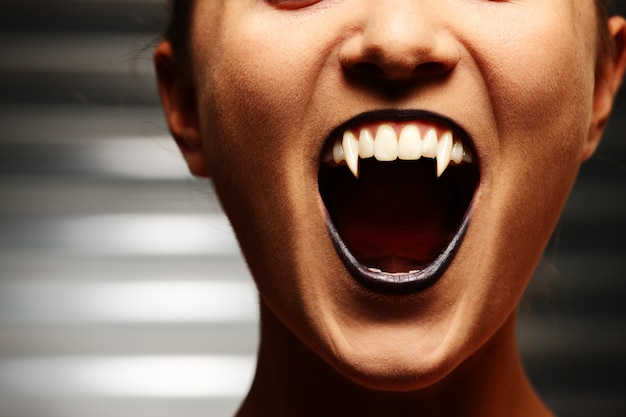The image portrays a striking, eerie close-up of what appears to be a younger woman's face, focusing from the lower edge of her eyelids down to the middle of her neck. Her skin has a slightly darker complexion, and her hair appears to be pulled back, with some wispy strands visible. The most defining feature is her wide-open mouth, revealing very sharp, white, vampire-like fangs, with a hint of reddish gumline beneath her lower lip. The woman wears black, possibly purplish, lipstick, and her lips are parted enough to see her tongue, suggesting she might be screaming or pretending to be a vampire. Her bottom eyelids have an orangish-red hue. Surrounding her face is a blurred background that seems metallic or like wide mini-blinds, with silver and dark gray tones on either side. The photo captures both of her ears and gives a slightly distorted appearance to her chin due to the exaggerated openness of her mouth.